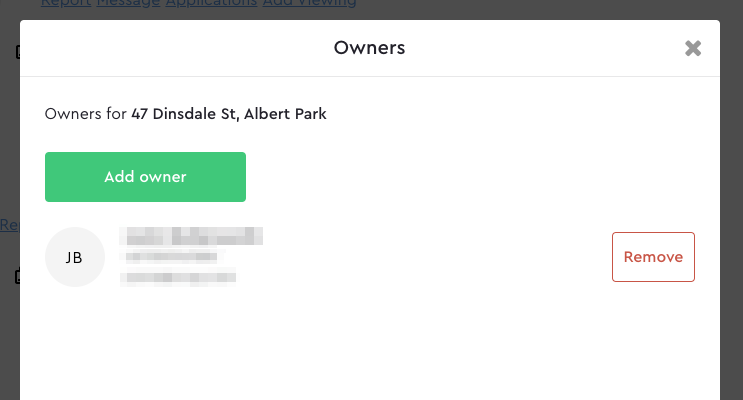The image displays a pop-up window with a black outline and a gray 'X' in the upper right corner for closing the window. The background of the pop-up is white. At the top, it reads "Owners for 47 Dinsdale Street, Albert Park." Below, there is a prominent green button with the text "Add Owner" in white. Listed under this text is the abbreviation "JB" in a gray circle next to some information that has been blurred. There is also a white rectangular button with a red outline and the word "Remove" in red text. The page features colors such as black, white, gray, green, and red. The bottom portion of the pop-up is cut off, indicating that there is more information that can't be seen in the image. The city or specific location details beyond "Albert Park" are not provided.